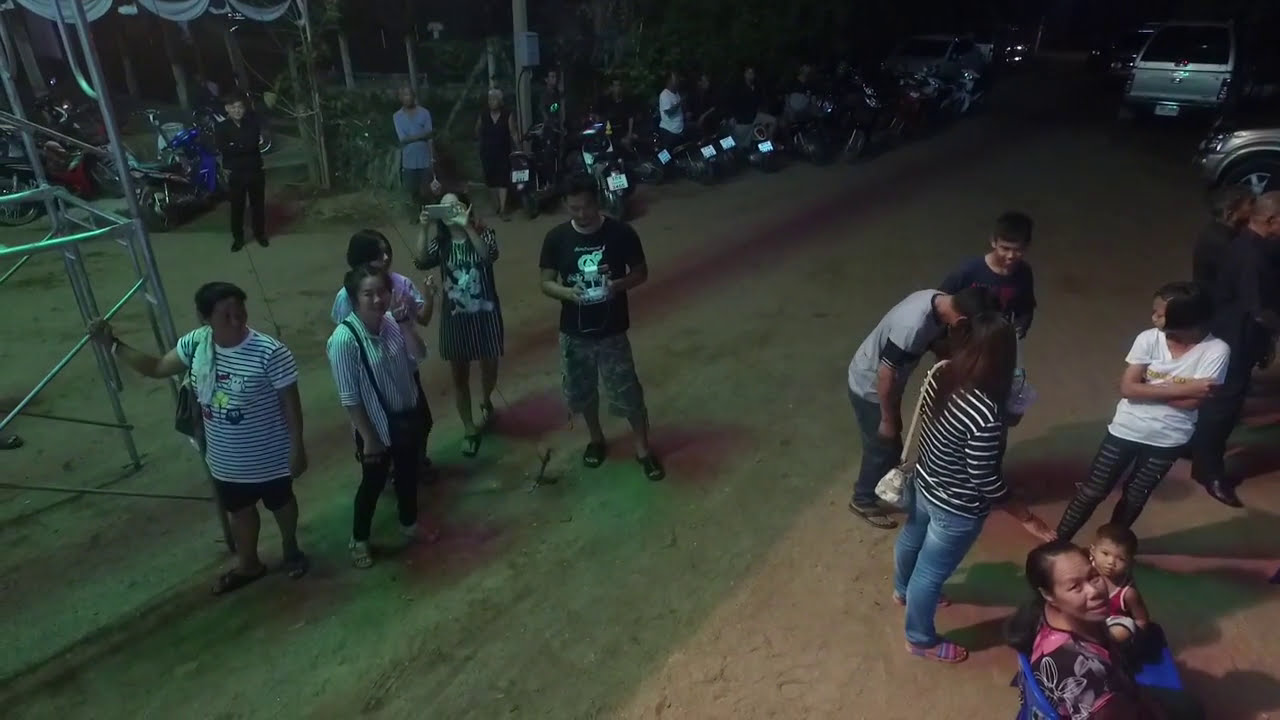The image captures a group of approximately 12 to 20 people standing around in a dimly lit, outdoor dirt lot. Taken from an elevated vantage point about 15 to 20 feet above, the photograph includes casual clusters of individuals who seem to be of Latino and possibly Asian descent, dressed in shorts, jeans, t-shirts, and blouses. In the center of the image, a standout woman holds a baby dressed in a jersey who both look directly at the camera. Scattered behind and around them are more people, some looking up towards the vantage point, likely in reaction to a drone being controlled by a man holding remote controls. Their shadows are cast towards the lower right corner, illuminated by an unclear light source leaving large portions of the scene in shadow, creating a somewhat dreary atmosphere. On the periphery, metal scaffolding can be seen to the left, along with several motorcycles, mopeds, and a couple of parked cars on the upper right, hinting at the scene's possible connection to an event or gathering.